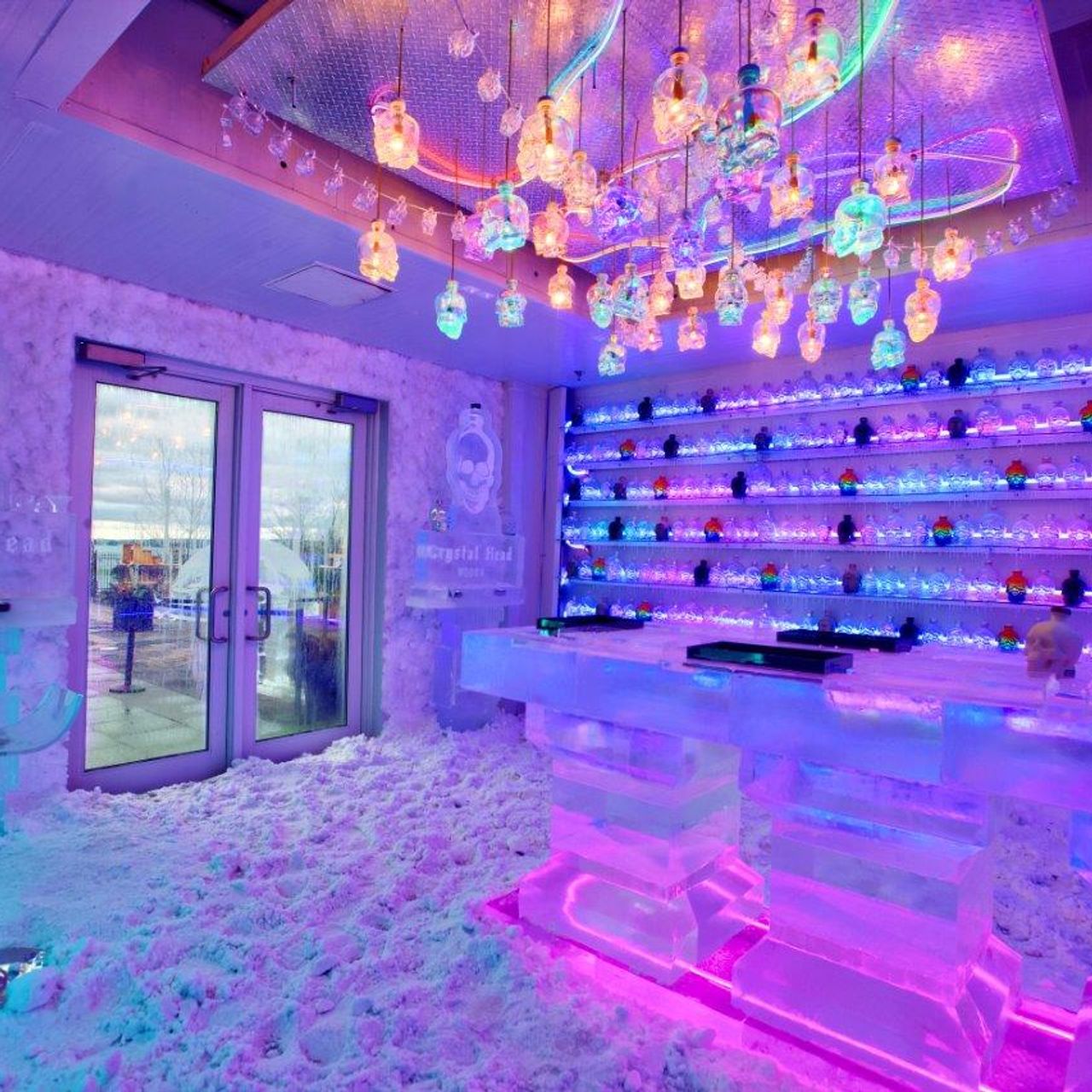This photograph depicts an intriguing bar setup that appears to be themed around ice and crystal elements, creating an ambience suggestive of a cold climate. The walls of the room are painted with a light purple hue, complemented by a pinkish and lavender glow cast from the overhead lighting, which features several orange and light green covers. The double glass doors at the back open to an outdoor scene with a typical sunny day atmosphere, characterized by blue skies and white clouds.

Inside, the entire floor is covered with a fluffy-looking substance resembling trampled snow. The central feature of the room is a bar that has a distinct icy appearance, as if constructed from large blocks of ice supported by ice pillars. The bar itself emits neon yellow and blue light from below, enhancing its translucent, icy look. Resting on this bar are three black rectangular items, as well as a glass or crystal skull, which might be part of an advertisement. This advertisement, placed near the doors, includes a text that reads "crystal head" beside a sculptural piece also shaped like a skull.

The back wall is lined with six shelves, hosting a variety of items that seem to be made from crystal or glass. These items are of myriad colors, including clear, dark, and rainbow hues, contributing to the overall vibrant yet chilly atmosphere of the room. Additionally, dangling from the ceiling are numerous single bulbs suspended at varying lengths, each housed within clear glass skulls, and exhibiting predominantly blue or orange hues. These elements together make for a visually striking and consistent theme throughout the bar, reminiscent of an ice palace or a high-end, crystal-themed lounge. Notably, there are no people present in the image, allowing the unique and detailed decor to fully capture the observer's attention.